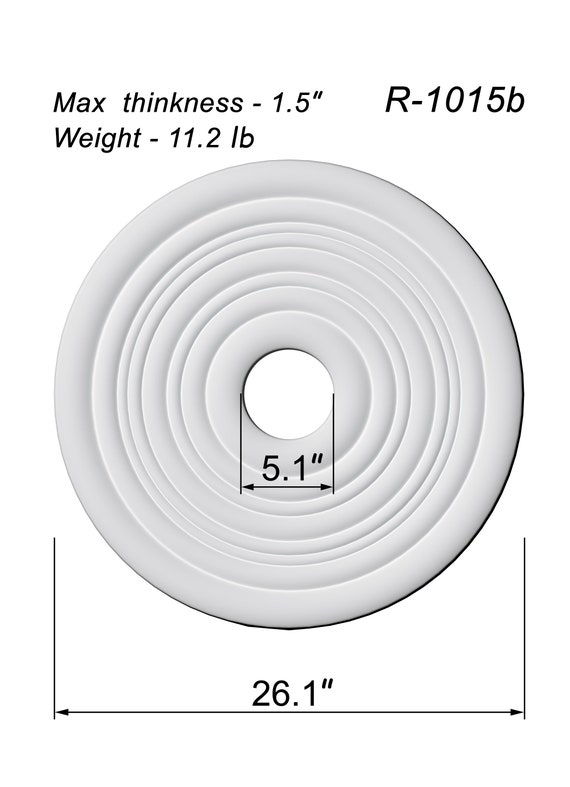This detailed diagram showcases a white disc composed of multiple concentric circles with varying widths. At the center of the disc is a hole, with arrows indicating its inner diameter of 5.1 inches. The outermost circumference of the disc measures 26.1 inches. The disc's maximum thickness is specified as 1.5 inches. It has a total weight of 11.2 pounds. The top of the image features the model number "R-1015B" in black font. Overall, this diagram meticulously details the disc's dimensions, thickness, and weight without any additional contextual information about its use.